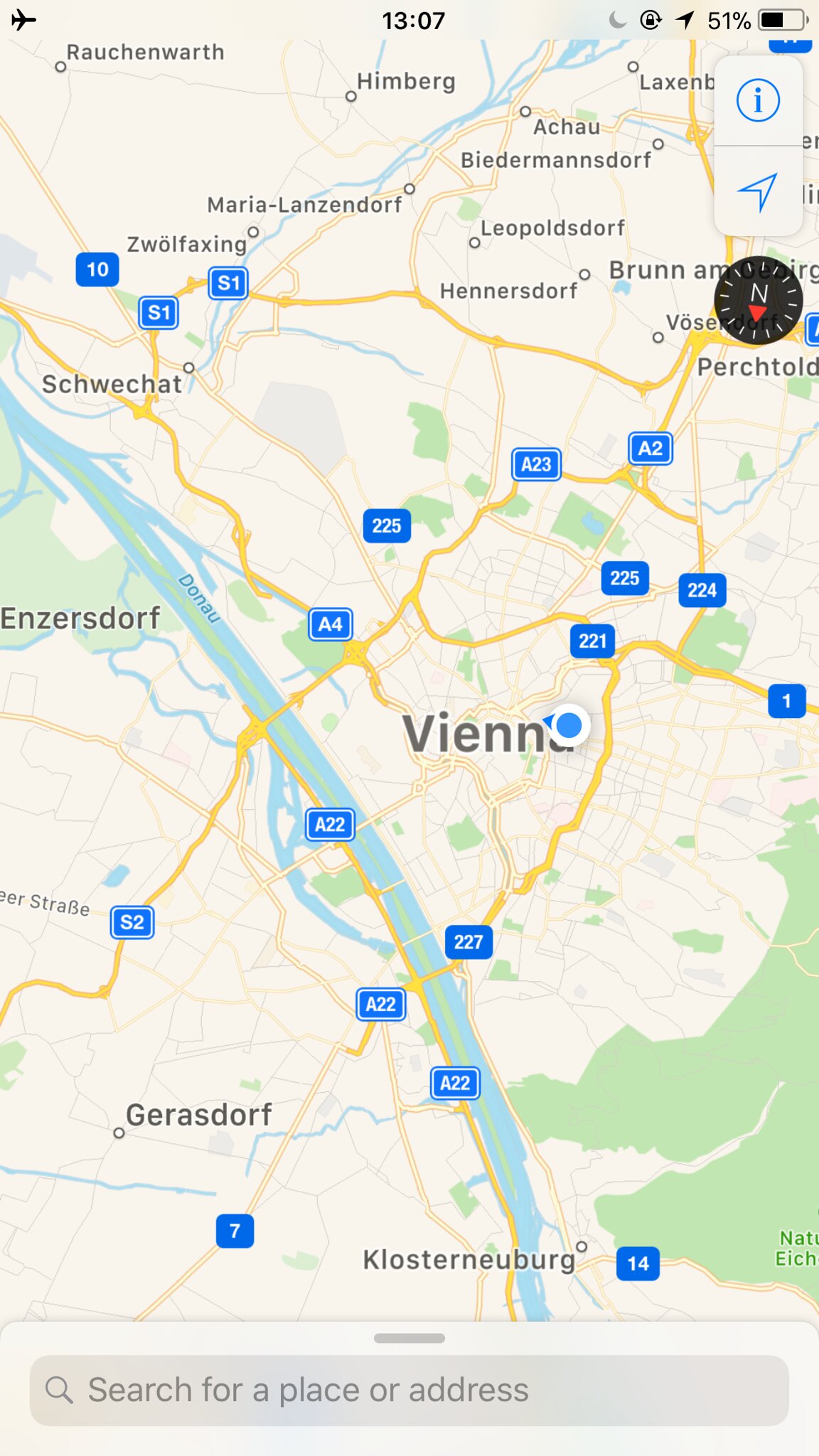The image showcases a detailed screenshot of a maps application focused on Vienna, Austria. At the bottom of the screen, there is a search bar with the prompt "Search for a place or address," inviting the user to input their destination. The map prominently features the Donau (Danube) River, which flows diagonally from the top left to just right of the center at the bottom. Several towns and cities are labeled, including Gerasdorf, Klosterneuburg, Schwächcat, Hennersdorf, Perchtoldsdorf, Leopoldsdorf, Achau, Biedermannsdorf, and Himberg.

Numerous routes are marked with blue rectangles containing white text, displaying designations such as A22, A23, A2, A4, 1, 227, 221, 224, and 225, indicating various highways and roads in the area.

The top-left corner of the display features an airplane mode icon, suggesting the device is not connected to cellular networks. The time is shown as 13:07, accompanied by icons for a moon indicative of a sleep mode, a padlock within a circle symbolizing security, a directional arrow, and the battery charge level at 51%. Additionally, a compass icon is situated just below the right corner, likely providing orientation for navigating the map.